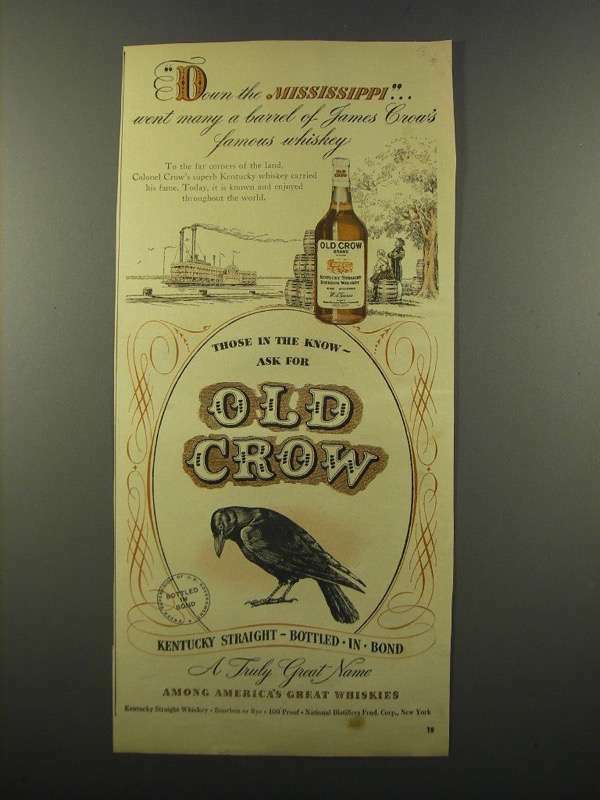This vintage advertisement for Old Crow bourbon features a weathered background with a dark olive-green hue, giving it an aged, nostalgic appearance. Dominating the center of the ad in an old-timey, saloon-style font, the words "Old Crow" command attention. Above this, it proudly proclaims "Those in the know ask for Old Crow." Beneath the brand name, an illustration of a black crow faces left, followed by the text "Kentucky Straight Bottled in Bond" encased in a ribbon design. The tagline, "A truly great name among America's great whiskeys," is prominently displayed below. 

The upper section of the ad sets a scene with the phrase "Down the Mississippi went many a barrel of James Crow's famous whiskey" in spirally lettering. Further text details how Colonel Crow's superb Kentucky whiskey reached the far corners of the land and is enjoyed worldwide today. Illustrations enrich the narrative: a riverboat meanders down the Mississippi River, with a figure seated on one of many barrels of Old Crow whiskey along the shore. In the foreground, a realistic image of an Old Crow whiskey bottle stands prominently. Decorative elements, such as an oval encircling parts of the text and crossed lines along the sides, add a touch of elegance. Additional fine print mentions the whiskey's 100 proof status and references its New York bottling. This ad exemplifies the brand's storied heritage and widespread acclaim.